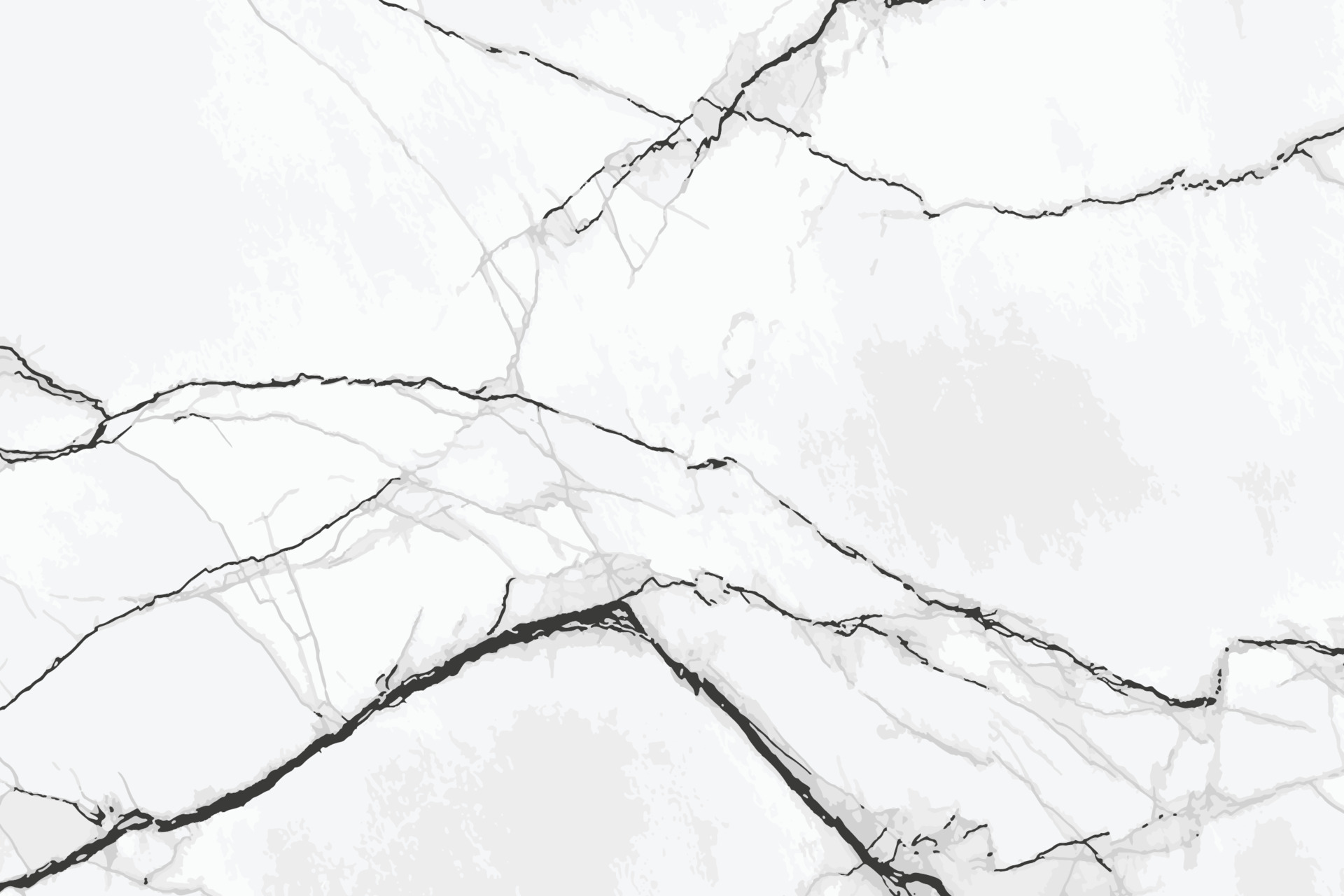The image appears to be a computer-generated representation of a light-colored marble surface, primarily in shades of white, black, and gray. It features a network of black and gray cracks traversing through a predominantly white and light gray background. One prominent black crack originates in the upper left corner, extends downward and to the right, crossing slightly past the center before continuing straight to the right edge. Another visible crack starts just right of center at the top, moves downward to the left, and intersects with the earlier crack. Additionally, two converging lines on the left side merge and proceed diagonally down to the right, eventually exiting the image on the right side. A darker line begins in the bottom left corner, ascends towards the middle, and then shifts downward and slightly to the right, ultimately disappearing off the bottom right edge. Scattered around these primary cracks are lighter gray fissures, adding depth and detail to the pattern, reminiscent of natural marble grain. The overall impression is of a close-up view of a marbled surface, showcasing its intricate crack formations, which could potentially be part of a larger structure like a sink or cabinet.